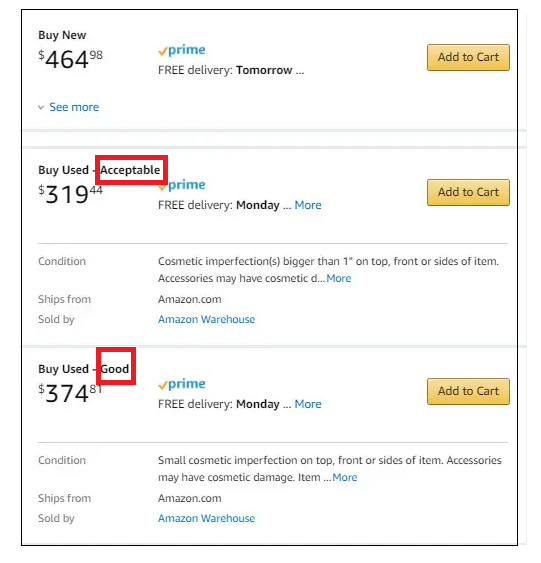Here's a more detailed and clean caption for the image:

---

The image displays a section of an Amazon product listing page, showcasing three different purchase options. The leftmost column presents the prices for each option, starting with the "Buy New" option at the top and followed by two "Buy Used" options below it. Each option is separated by horizontal line dividers.

Adjacent to the prices in the middle column, the Amazon Prime logo with a yellow check mark and blue "Prime" text is prominently featured, indicating the availability of Prime benefits. Below the logo, the delivery expectations are presented: "Free delivery tomorrow" for the "Buy New" option, "Free delivery Monday" for the first "Buy Used" option, and another "Free delivery Monday" for the second "Buy Used" option, each with a link for more details.

On the right side of the image, there's a yellow "Add to Cart" button with black text, aligned with each purchase option, allowing users to easily add the desired product to their cart.

---